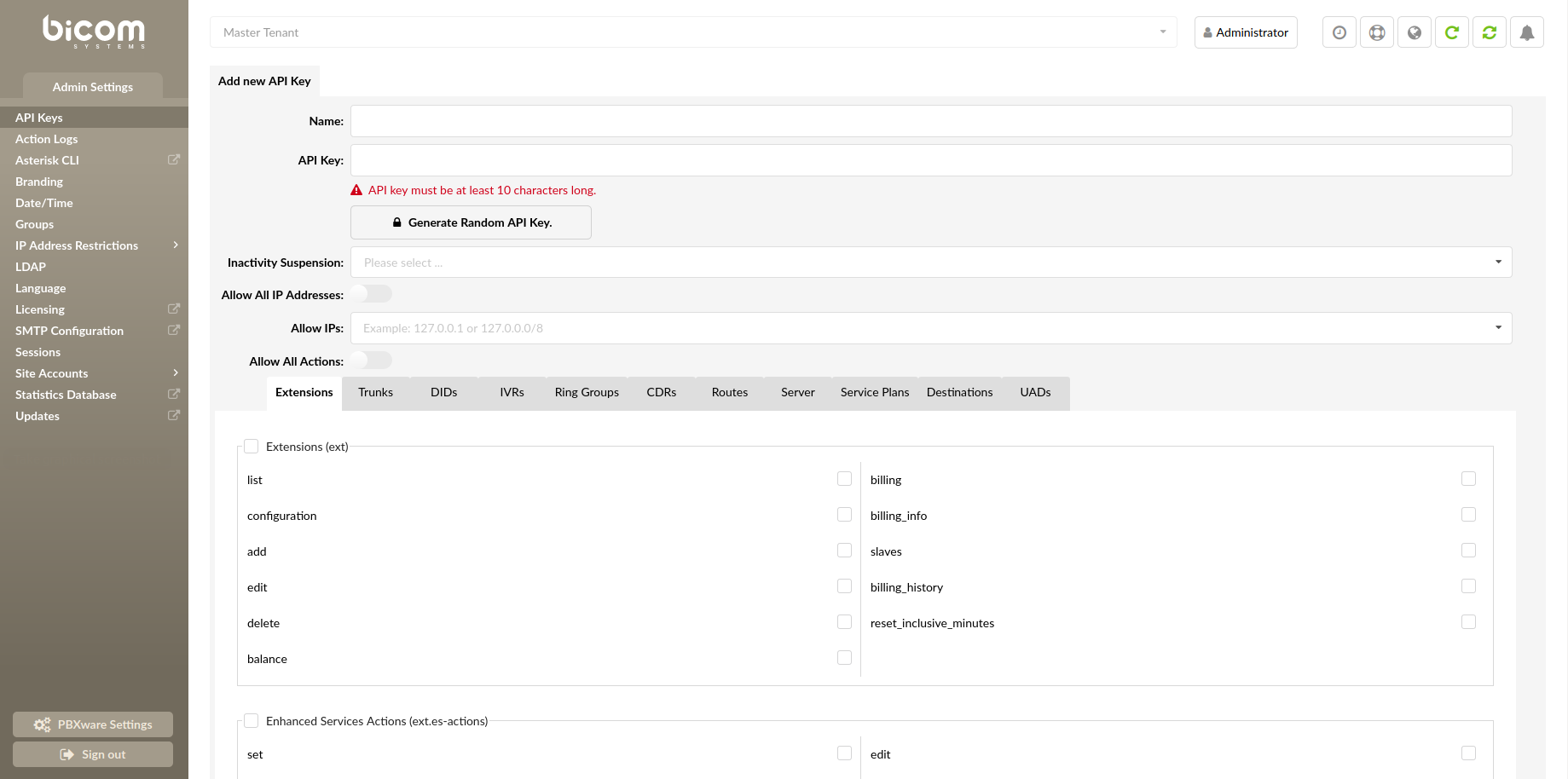The image depicts a settings interface for a platform called Bicom. While not exactly a traditional webpage, it appears more like an administrative dashboard dedicated to managing various configurations. The majority of the text on the page is notably small, making it challenging to read. Key elements visible include options to manage API keys, with fields for entering new keys, names, and the actual key itself. However, no values have been entered into these fields as of yet.

Additional settings visible on the interface include "Inactivity Suppression" and "Allow IPs," which likely serves as a whitelist feature for authorized users. The left pane, styled in a bronze color, provides navigation to other sections such as Action Logs, CLI, Branding, Date & Time configurations, Groups, and more, suggesting comprehensive network access management capabilities.

At the top right corner of the page, there are several prominent buttons, one labeled "Administrator," which likely leads to more options or settings, and others including a refresh icon and an alarm icon, the latter presumably for notifications or alerts. The overall interface has a clean, predominantly white background, which contrasts with the bronze-colored navigation pane on the left, giving it a structured yet user-centric appearance.